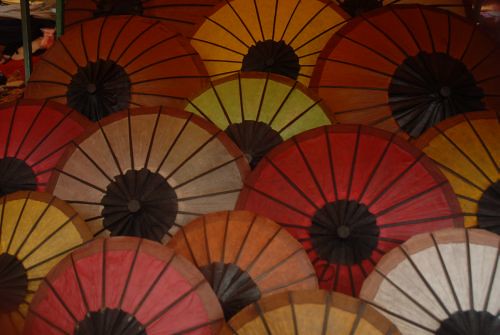The image displays an array of umbrella tops, covering the entire frame with each umbrella open and oriented downward, as if viewed from above. The umbrellas, approximately 30 to 50 percent wider than they are tall, feature a striking design with a central black dot from which black spokes emanate, giving them a somewhat floral appearance. These umbrellas come in a variety of colors, including shades of yellow, orange, red, pink, white, tan, and off-white, each adorned with a light brown rim around their edges. The array of umbrellas fills the image densely, arranged in rows of three to four per row, with the exception of the upper left corner, where part of two black beams or bars are visible, along with what appears to be the bottom of a metal chair's legs. The vibrant colors and oriental designs create a visually captivating pattern, accentuated by the consistent black elements at their centers.